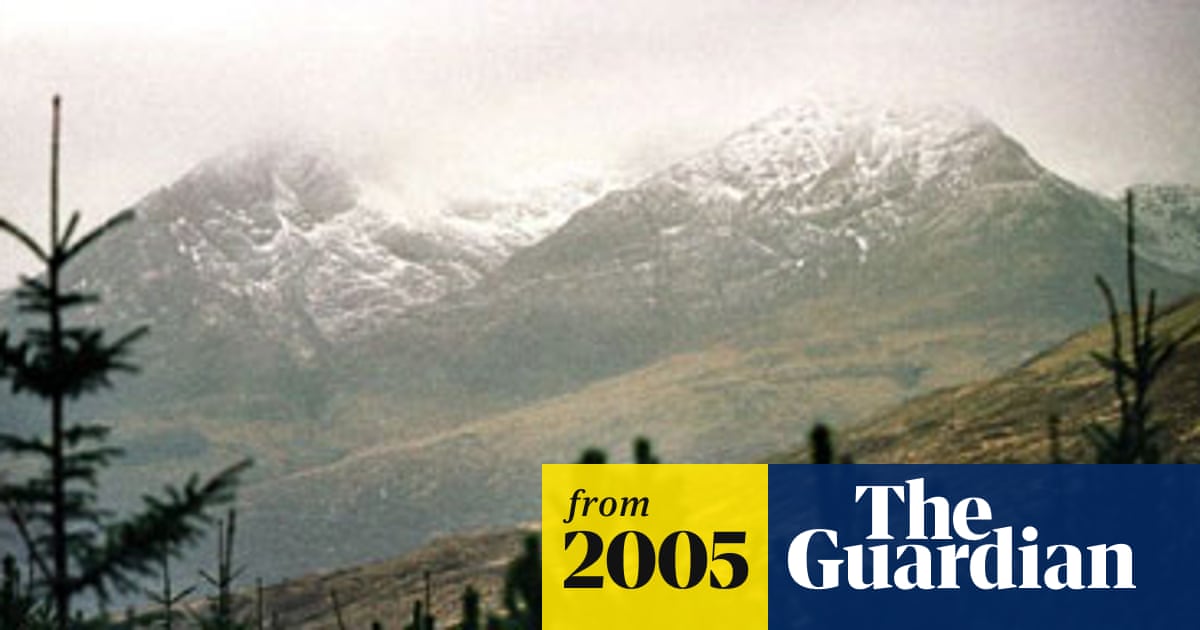This image, likely extracted from a 2005 issue of The Guardian, showcases a breathtaking mountainscape. In the far background, two prominent snow-capped mountains are seen fading into the sun or the clouds on a cloudy day. The foreground reveals another mountain without snow, dotted with evergreen and pine trees, their tops bare but lush from the middle downwards. The composition suggests it could be taken from a high vantage point, perhaps within a state park, capturing both the majestic, snow-covered peaks and the wooded hillsides below. The caption "From 2005, The Guardian" in yellow and blue text graces the bottom right corner, indicating its origin from a reputable publication, possibly a magazine, newspaper, or book.